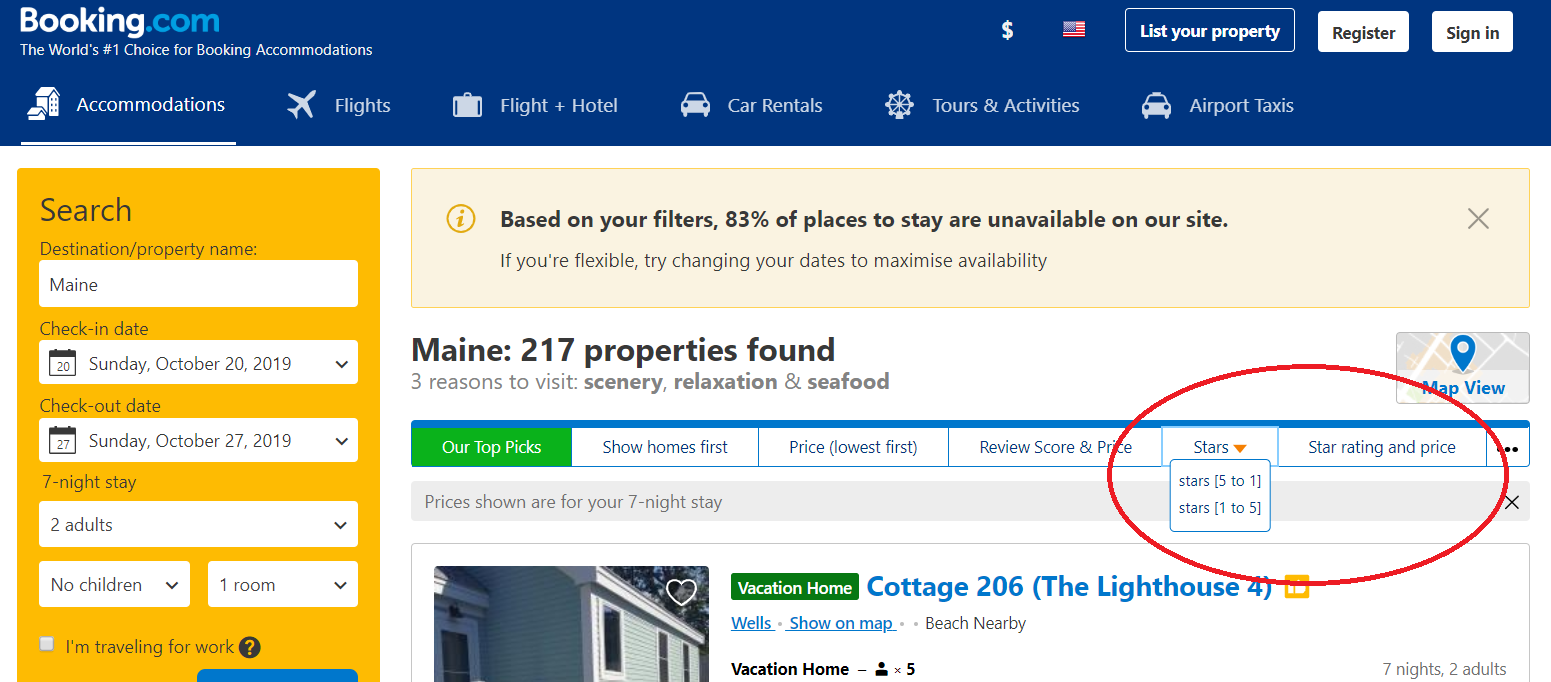A screenshot captured from a computer screen, likely a laptop or desktop given the long rectangular cropping, showcasing the homepage of Booking.com. At the very top of the page, a dark blue navigation bar prominently displays the Booking.com logo. Adjacent to the logo is a set of controls featuring a dollar sign, the American flag indicating the US region, an option that prompts users to list their property, and two buttons labeled "Register" and "Sign In."

Beneath the navigation bar, a tagline reads, "The world's number one choice for booking accommodations." Directly below, a horizontal menu with corresponding icons lists various booking categories: Accommodations, Flights, Flight + Hotel, Car Rentals, Tours & Activities, and Airport Taxi.

At the center of the page, a search bar reveals a query for accommodations in Maine, with specified check-in and check-out dates from Sunday, October 20th, 2019 to October 27th, 2019. The search results indicate that 217 properties have been found for the specified dates in Maine.